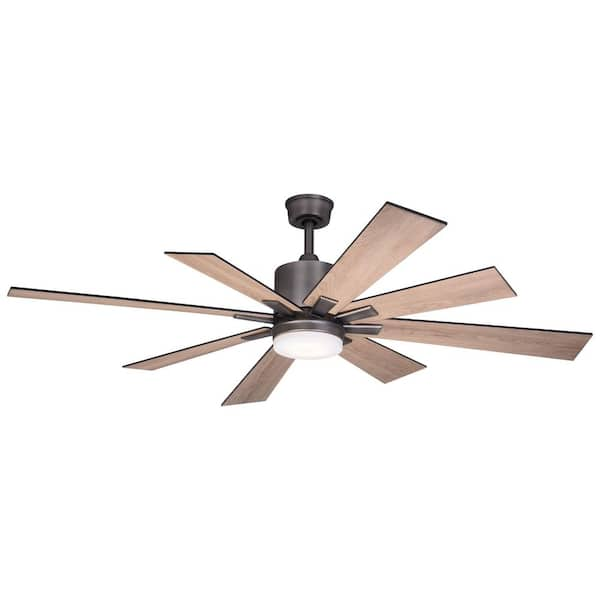A stylish ceiling fan with a unique design, featuring eight square brown blades connected to a dark brown, cylindrical center. The fan's center is supported by a slender, round base atop a narrow post. Matching dark brown brackets secure the blades to the body. There is a round white light fixture affixed to the underside of the fan, providing soft illumination. The eight blades are arranged in two distinct layers: the upper layer consists of four shorter blades forming an 'X' shape, while the lower layer includes four longer blades forming a '+' shape. The longer blades, which extend from front to back and left to right, appear more prominent than the diagonal shorter ones, giving the fan a dynamic and visually engaging appearance.